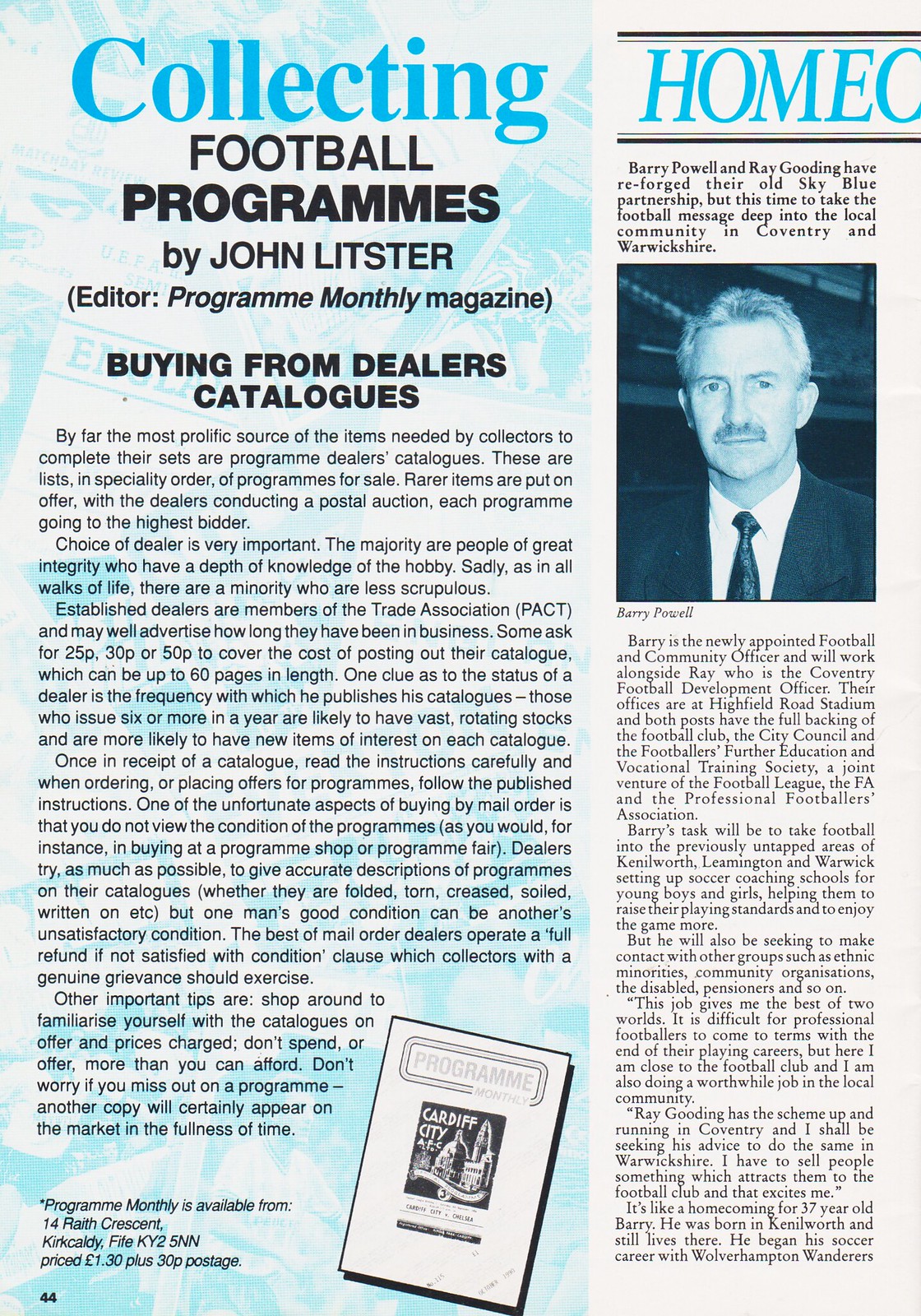The image depicts a newspaper clipping divided into two distinct columns. The left column, which occupies two-thirds of the picture, features a blue and white background and prominently starts with the word "Collecting" in blue letters. Beneath it, the heading reads “Football Programs by John Litster” followed by “Editor, Program Monthly Magazine” in brackets. Below, a bold title states “Buying from Dealers' Catalogues,” leading into several paragraphs of detailed text. At the bottom of this column, there's a mention that "Program Monthly is available from 14 Wraith Crescent, Kirkcaldy KY2 5NN, priced £1.30 plus 30p postage," along with a sketch of a catalog cover that appears to feature an illustration of a castle. On the right column, which has a cream background, the text starts with "Homeo" (with the rest cut off in the image). Beneath this, there is a black and white photograph of an older man named Barry Powell, dressed in a suit and tie, and featuring a mustache. The image shows his head and shoulders. Underneath Barry Powell's photograph, there is an extensive biographical text about him.